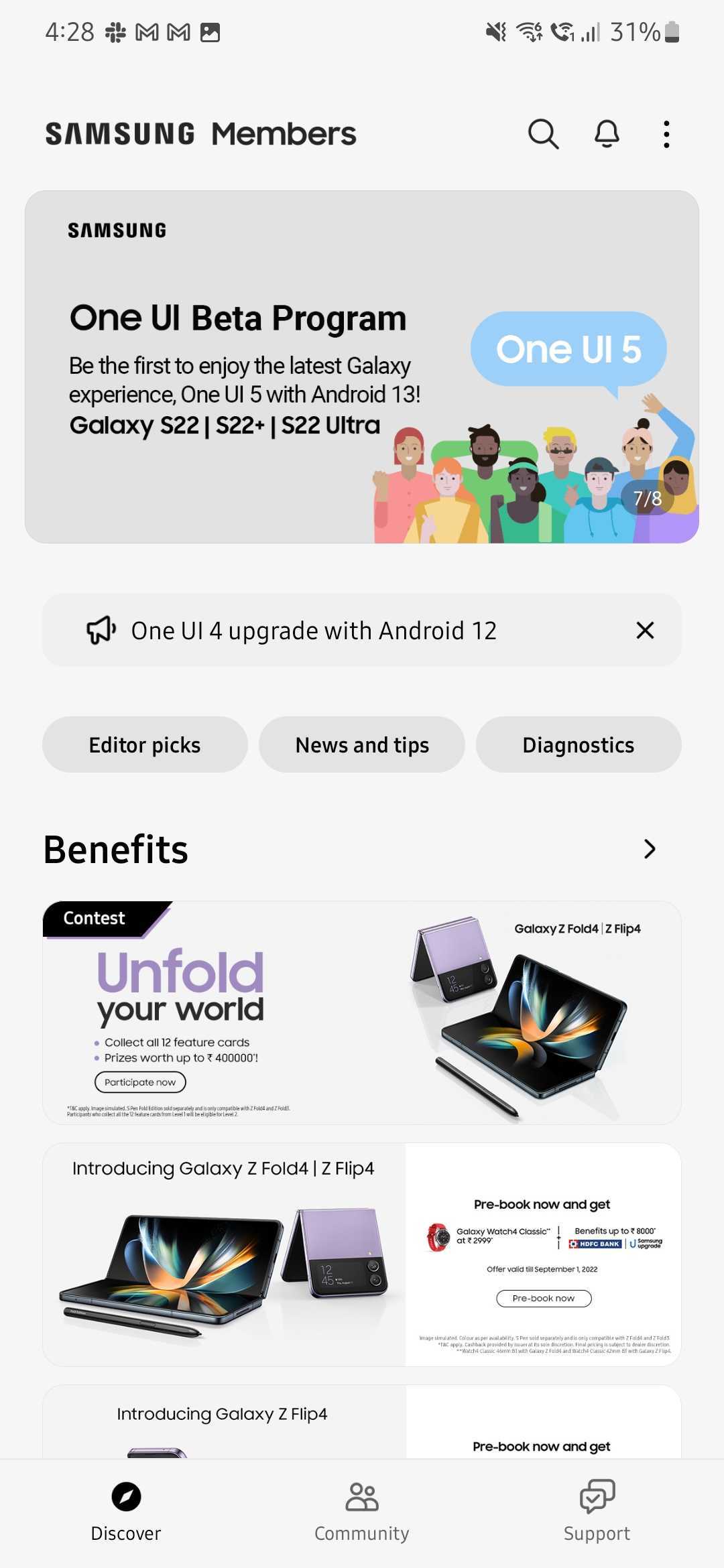The image displays a screenshot of a Samsung email opened on a smartphone. The top section of the phone screen shows the standard time and various phone status icons. Below that, the email is identified as being from "Samsung Members."

A prominent gray box beneath the header contains an announcement about the One UI beta program. The text within the box invites users to "Be the first to enjoy the latest Galaxy experience: One UI 5 with Android 13." Below this announcement, it lists compatible Samsung models, specifically the Galaxy S22, S22+, and S22 Ultra. 

To the right of this text, there are colorful illustrations of various characters wearing red, yellow, green, blue, and purple shirts. One of the characters has a speech bubble that reads, "One UI 5." Below the characters, another text line announces "One UI 4 Upgrade with Android 12."

Further down the screen, three buttons are displayed for navigating different sections: "Editor's Picks," "News and Tips," and "Diagnostics." Below these buttons, there is a section labeled "Benefits," which features images of phones including the Galaxy Z Fold and Z Flip 4. The phones are shown in both folded and unfolded states, along with a stylus. Accompanying this display is a pre-booking offer which mentions "Pre-book now and get" something resembling a small watch, though it is quite small and hard to see clearly.

At the very bottom of the email, there are links to "Discover," "Community," and "Support."